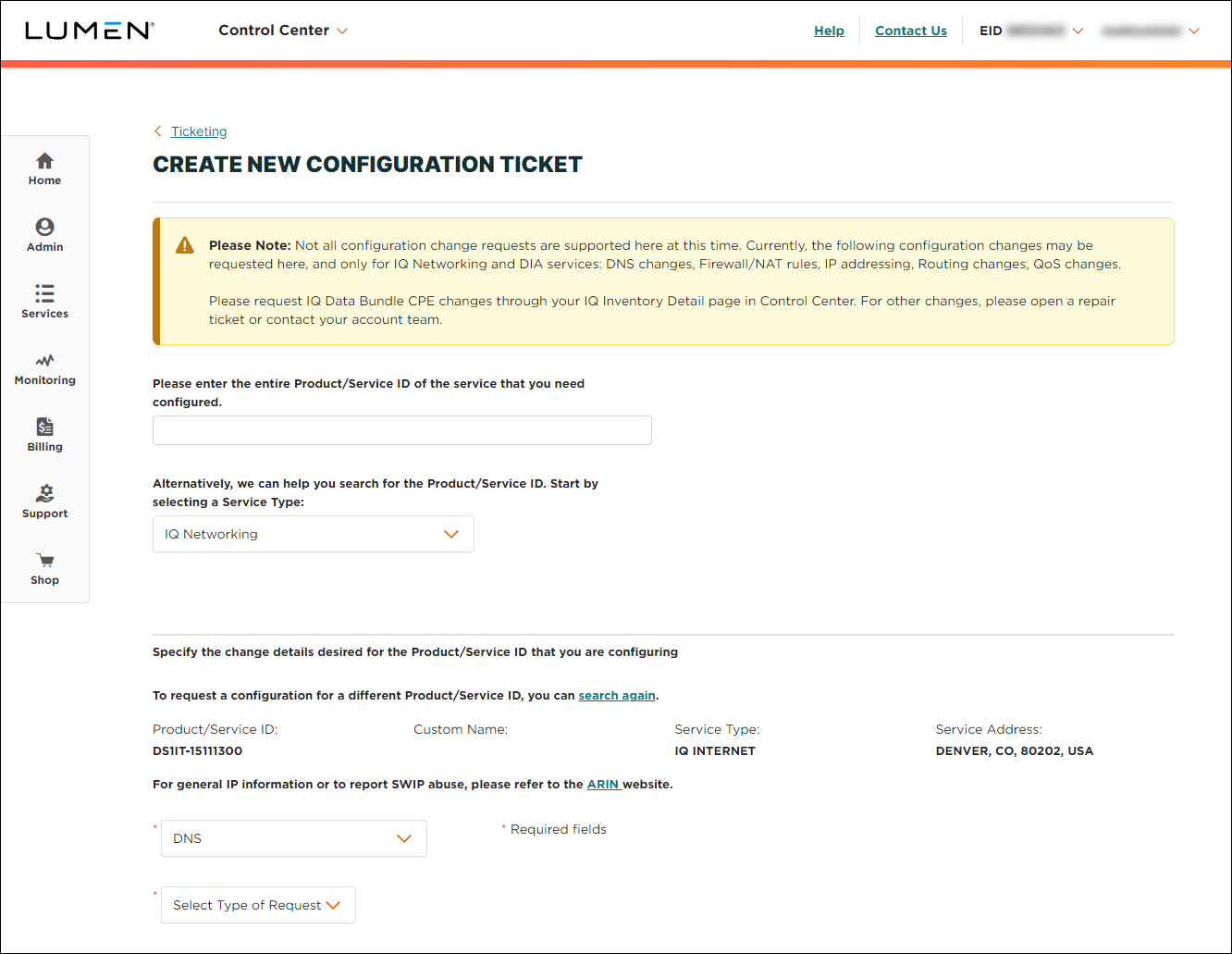Screenshot of the Control Center Interface in the Lumen Program

In this detailed interface screenshot of the Lumen Control Center, the program name "Lumen" is prominently displayed in the upper left corner, followed by "Control Center." On the far right, "EID" is visible with certain areas blurred for privacy. The options "Explore Lumen," "Help," and "Contact Us" are listed in white print within a blue-bordered section on the right-hand side.

Running vertically along the left side of the interface is a gray-bordered menu featuring the following options: "Home," "Admin," "Services," "Monitoring," "Billing," "Support," and "Shop." The "Support" option is highlighted in blue, indicating it is currently active. The main content under "Support" displays the section titled "Ticketing," with a prompt to "Create New Configuration Ticket."

A prominent orange caution box featuring a triangle caution logo warns users: "Please note not all configuration change requests are supported here at this time. Currently, the following configuration changes may be requested here and only in IQ Networking and DIA services: DNS changes, firewall NAT rules, IP addressing, routing changes, QoS changes. Please request IQ bundle CPE changes through the IQ inventory detail page in the Control Center. For other changes, please open a repair ticket or contact your account team."

Further guidance is provided: "Please enter the entire product service ID of the service you need configured. Alternatively, you can help search for the product service ID by selecting a service type (IQ Networking) in a drop-down menu. Specify the change details desired for the product service ID that you are configuring. To request a configuration for a different product service ID, you can search again."

A sample product service ID, "DS1IT15111300," is provided, indicating "IQ Internet" as the service type, with the service address listed as Denver, Colorado 80202, USA. For general IP information or to report SWIP abuse, directions are given to refer to the ARIN website. The interface displays drop-down menus for "DNS" and to "Select Type of Request."